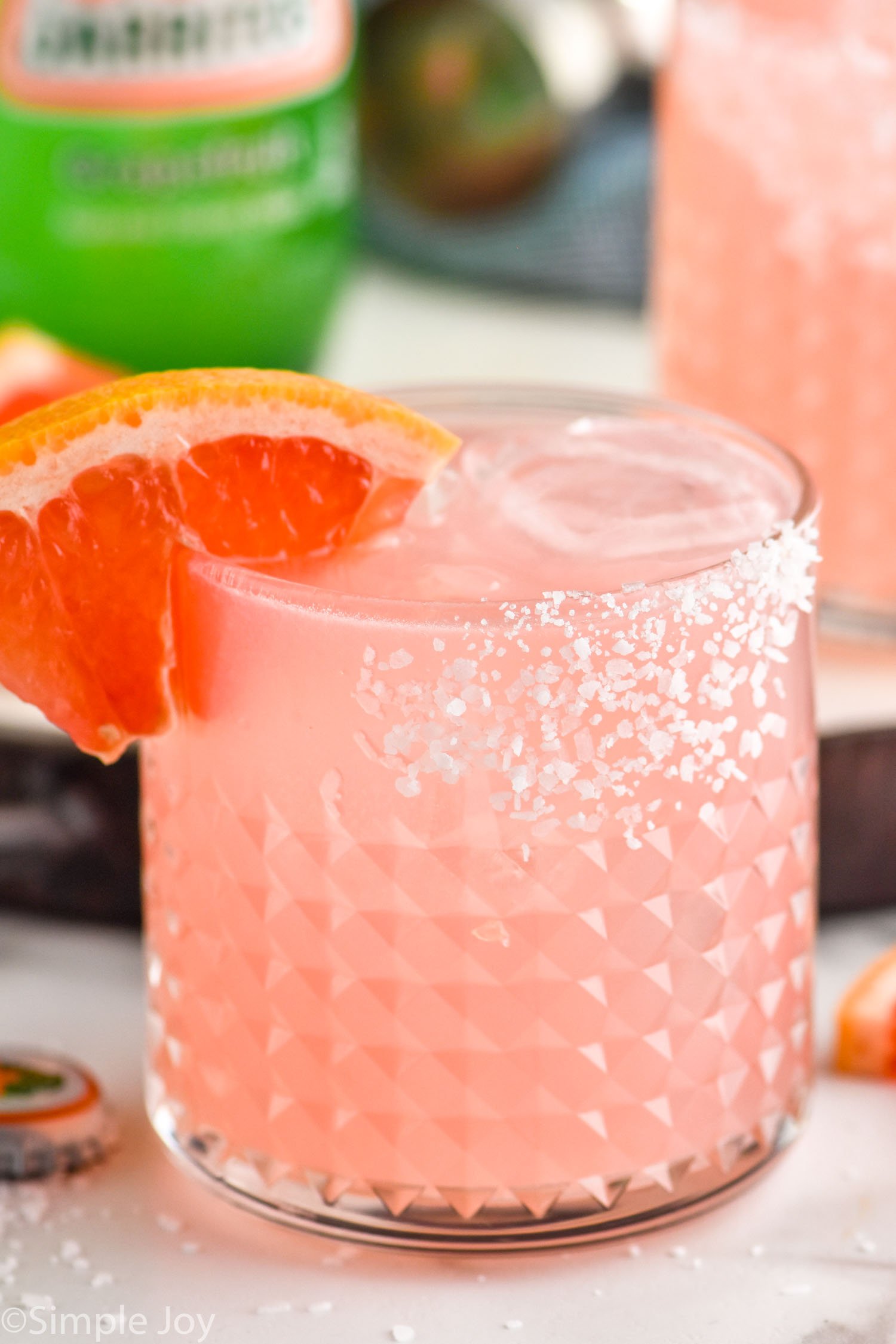The image features a close-up of a cocktail in a clear, textured tumbler glass with a pattern of bumpy squares extending two-thirds up from the bottom. The beverage is a light pink color, reminiscent of salmon, filled nearly to the rim with ice cubes visible inside. An orange slice, possibly a mandarin or tangerine, is perched on the left side of the glass, while salt or sugar coats the right side of the rim and extends down about a quarter of the way. The same salt or sugar is scattered on the white marble benchtop beneath the glass. To the left of the main glass is a discarded bottle cap, and an orange plastic object sits on the right. In the background, we can see a green bottle with blurred orange and white text and logo, suggesting it might be a soda bottle. Another similar glass containing the pink liquid is visible on a brown stand to the right, alongside a bottle lying on its side. The background is out of focus, drawing attention to the intricately textured glass, the vibrant pink drink, and the detailed garnish of the cocktail.